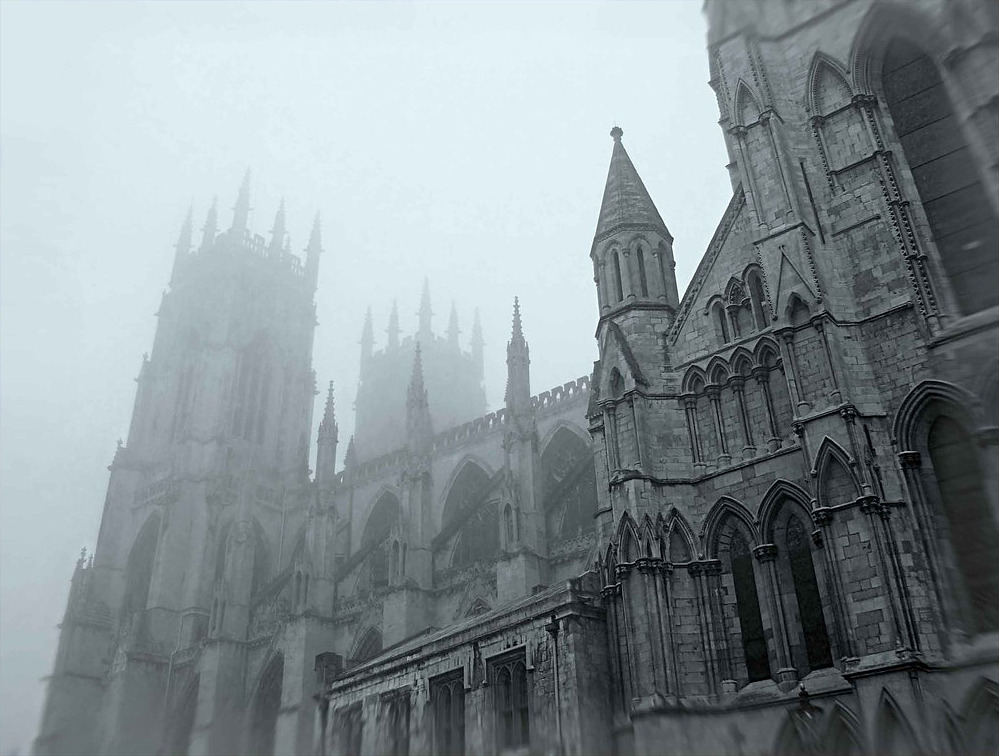This photograph showcases a grand, Gothic cathedral enveloped in a heavy fog, rendering the left side of the image particularly obscured. The scene captures an overcast, somewhat ominous atmosphere, with gray stonework blending into the grayscale tones of a pale blue, fog-filled sky. Rising up from the lower right corner, the cathedral dominates the frame with its ornate architectural features. The structure boasts numerous severely arched windows, intricate ornamentation, spires, and minarets that evoke a blend of Renaissance and Gothic styles, reminiscent of Notre Dame with its twin towers. These towers, along with the rest of the cathedral, become progressively fainter as they recede into the mist, lending a hauntingly ethereal quality to the image.